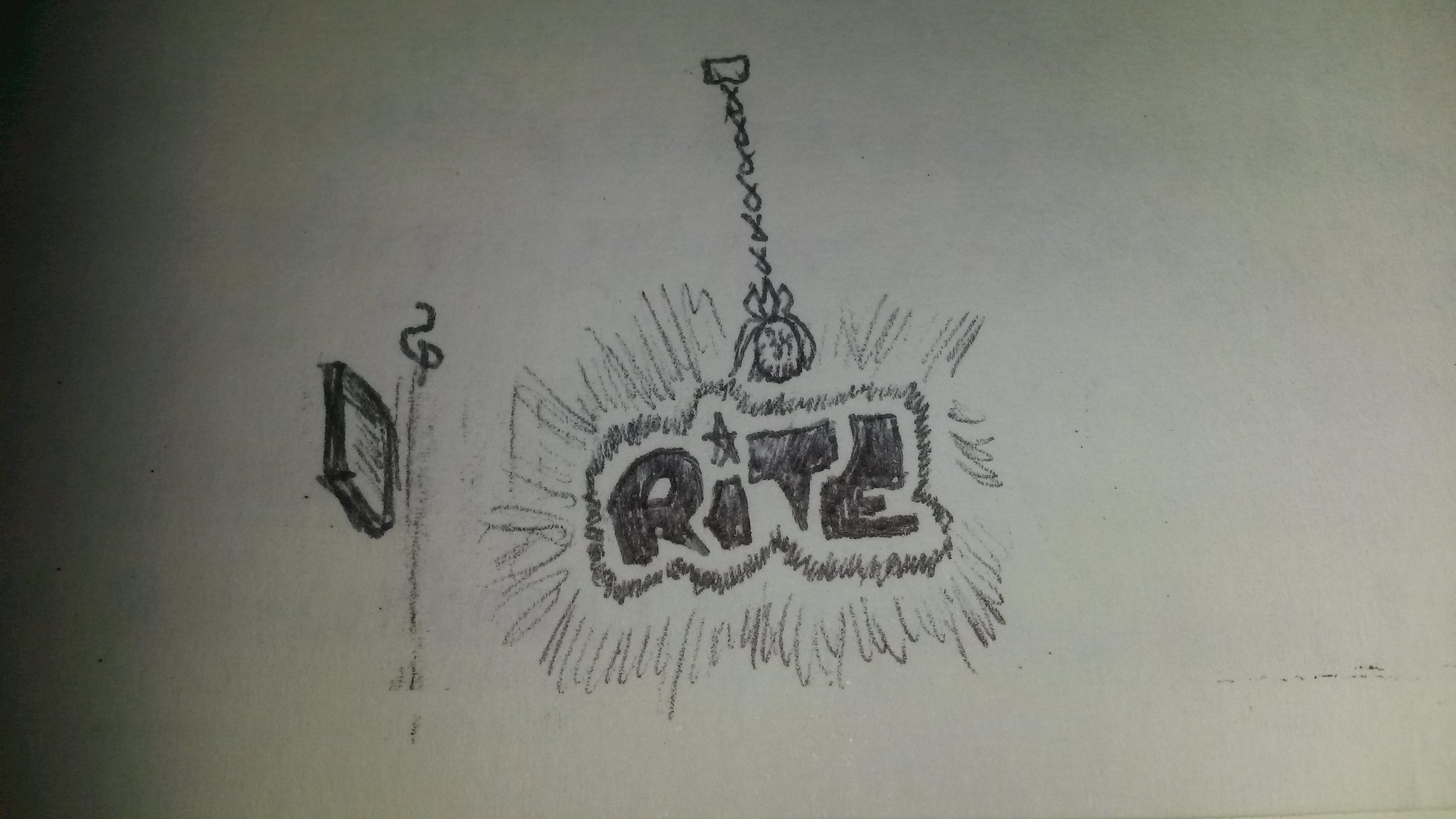This drawing features a central emblem with radiating lines arranged in a circular pattern. At the core of this emblem, the word "R.I.T.E." is inscribed, and above the letter 'I' is a star. A chain descends from above the letter 'T,' culminating in a small bag that appears to be floating above it. To the left of this central design is a long black line topped with a backward 'S,' and to its left, a black square diamond shape is visible. The entire artwork is drawn on a white piece of paper, with a faint shadow cast along the left edge. The letters in "R.I.T.E." are uniquely stylized with a jagged outline; the 'R' and 'T' have pointy bottoms, while the 'E' features an exaggeratedly large top and a slender bottom.